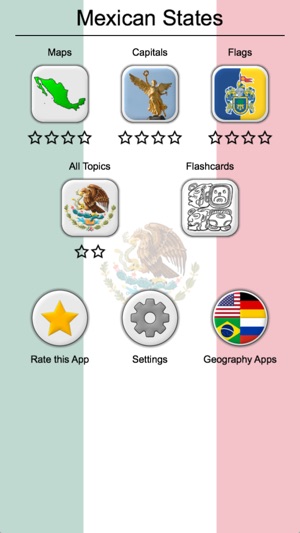In this image, the background is a vibrant Mexican flag, featuring three vertical stripes: green on the left, white in the middle, and red on the right. Centrally placed in the white stripe is a brown emblem resembling a bed.

The top section of the image prominently displays the words "Mexican State," indicating that the image pertains to the states of Mexico. Toward the top left corner, the label "maps" is displayed alongside a green map set against a grey square background. Above this map, the word "map" is written. Just below, there are four black stars intended for rating, though they are not colored in.

In the top center, the word "capitals" is written above a gold icon resembling a stage, which also lacks a rating. To the top right, the label "flags" is followed by an image of a flag that is blue on the right side and yellow on the left, incorporating an inner flag that is red.

Below these elements, there is a section labeled "flash card," featuring a white background with a black drawing. On the left side of the image, it says "all topics," accompanied by an icon of Mexico and a two-star rating.

At the bottom of the image are three buttons. The center button, labeled "settings," is grey. The bottom-left button says "rate this app," highlighted by a yellow star. The bottom-right button, labeled "geography apps," displays four flags: 
- The flag of the USA, which is red, white, and blue.
- The flag of Germany, which is red, yellow, and black.
- The flag of France or the Netherlands, which is white, blue, and red.
- The flag of Brazil, which is green, yellow, blue, and white.